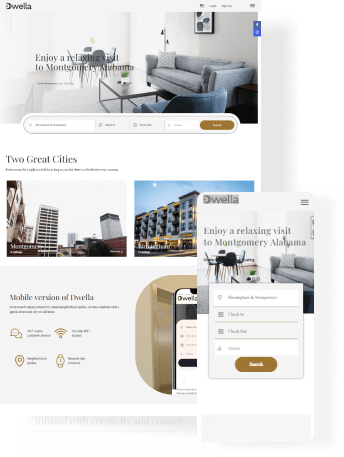This image, seemingly from a company named Dwella, features multiple elements. 

In the upper section, the company name "Dwella" is displayed in small text. The main visual is a photograph of a living room. The living room includes a gray couch positioned against light gray walls with a single framed picture hanging above it. The room also features a chair and a coffee table. An attempt to include a tagline, reading "Enjoy a relaxing visit to Montgomery, Alabama," is made within this setting. However, the tagline is difficult to read because it is rendered in a color that closely matches the furniture.

Adjacent to this, there are images of two cities with skyscrapers. The city on the left has a gray sky, while the city on the right showcases a blue sky. 

In the next part, a pop-up mentions "Dwella, Enjoy a Relaxing Visit to Montgomery, Alabama," suggesting this is the suggested tagline. This text could be more readable if moved up to the gray wall area.

Below this section, there's a brown drop-down box with a submit button. Additionally, there is information about a mobile version of the Dwella website, accompanied by a partial image of a cell phone. 

The design implies an interactive feature with a colored key, which might aid users in navigating or engaging with the content. Notably, the visual design decisions, such as color choices and text placement, could benefit from adjustments to improve readability and user experience.